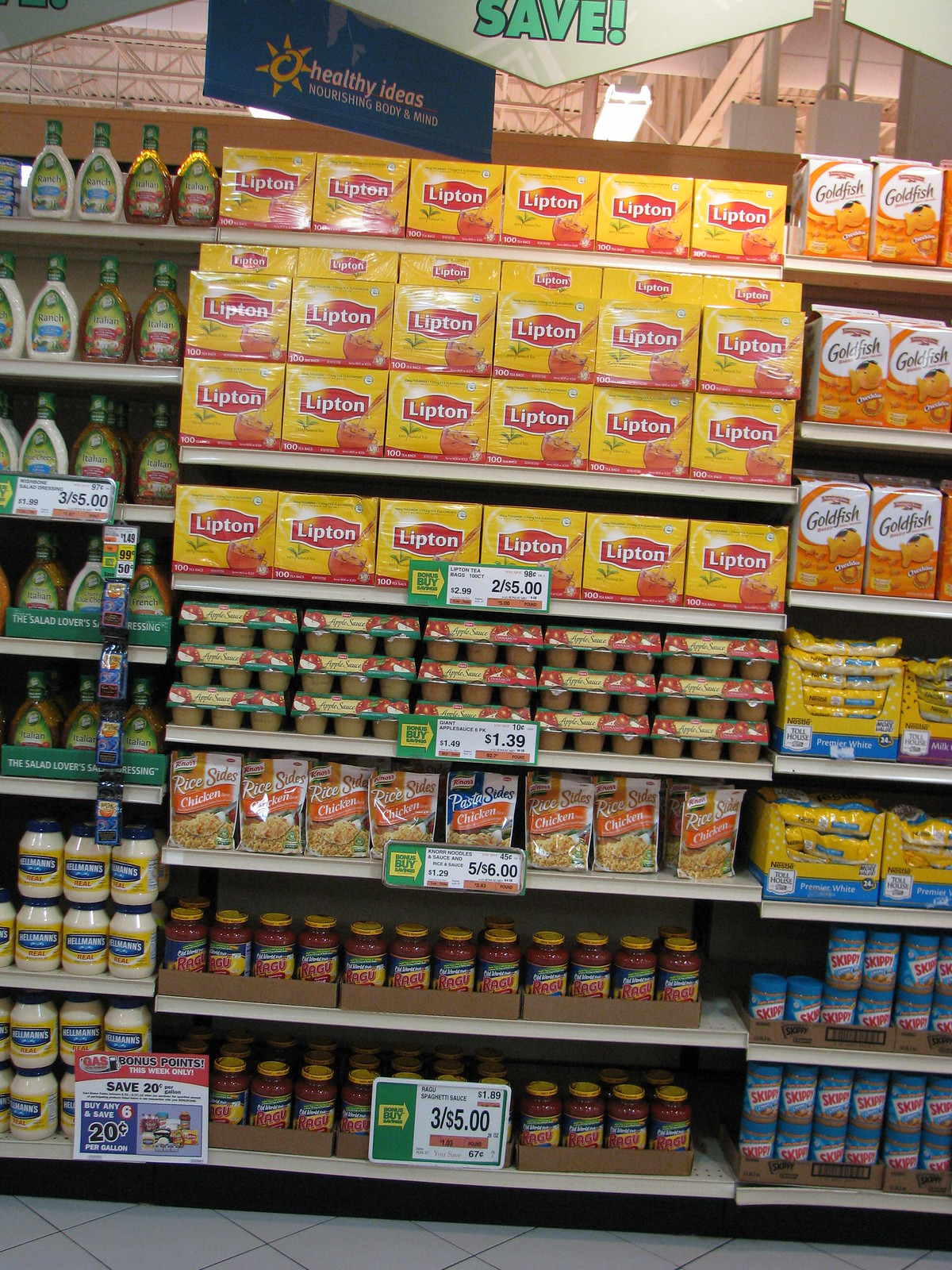The image depicts a section of a supermarket aisle showcasing an eclectic mix of products on white shelves, predominantly under special discount, as indicated by price tags in dollars. Dominating the middle section is a prominent display of Lipton iced tea in yellow boxes, occupying four shelves from the top. Directly below, one shelf is stocked with applesauce containers, followed by a shelf containing chicken rice packaging. Further down are two shelves brimming with varieties of pasta sauce. To the left of this central display, the top five shelves contain different types of salad dressings, while the bottom two shelves are stacked with Hellmann's mayonnaise. On the right side, three shelves are filled with large packages of Goldfish crackers, followed by two shelves with yellow packages of presumably rice, and beneath these, two shelves are dedicated to Skippy peanut butter, neatly stacked. The store’s ceiling features signs like a blue rectangular one stating "Healthy Ideas" with a sun logo and a slogan, "Nourishing Body and Mind." Additionally, a cream-colored arrow-shaped sign with "SAVE" in mint green is notable among the suspended signage. The overall color scheme of the products and signage includes vibrant yellows, oranges, blues, and greens, amidst the store’s exposed white ceiling.